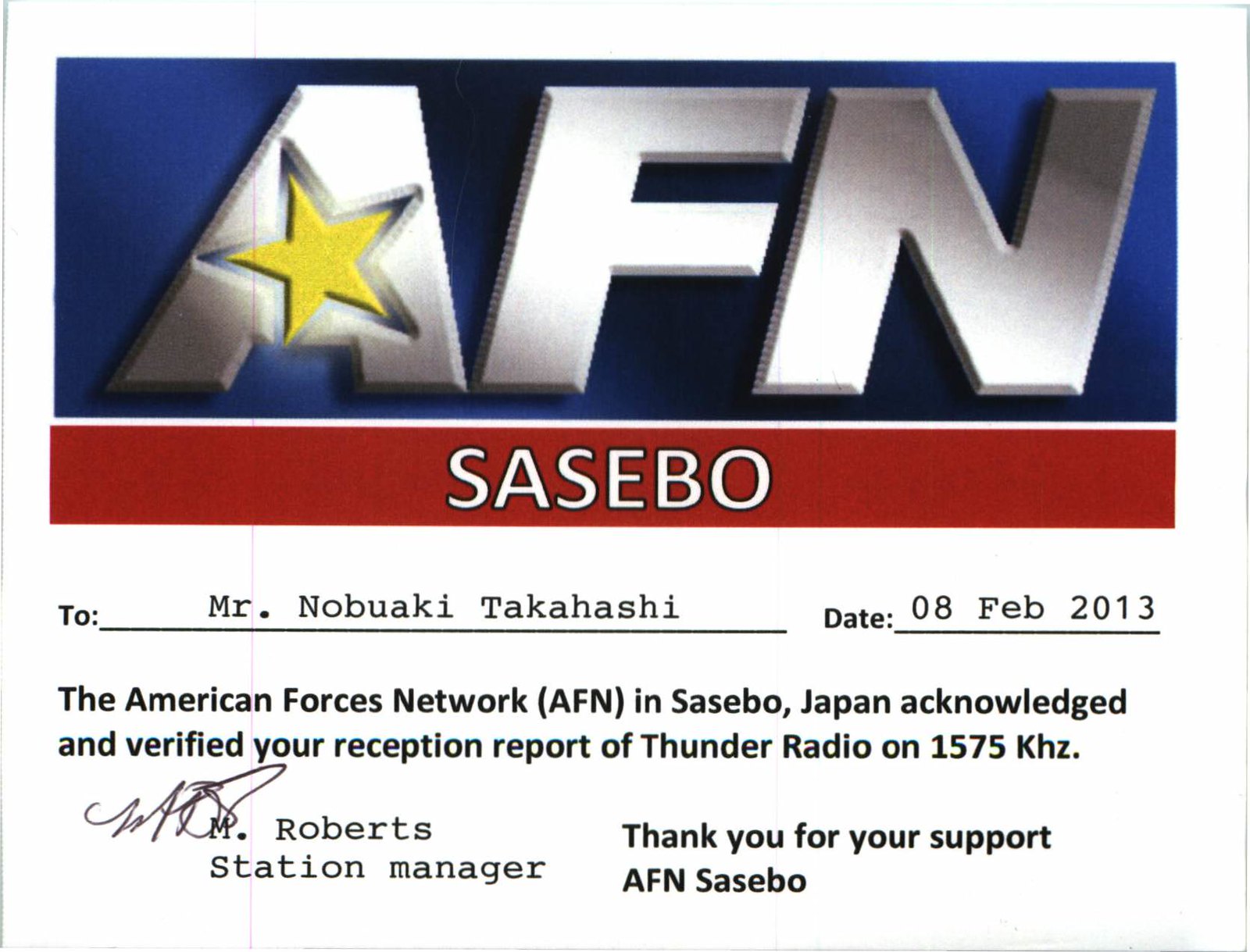The image depicts a confirmation certificate from the American Forces Network (AFN) in Sasebo, Japan. The white background features a prominent blue emblem in the upper half with white lettering spelling out "AFN." Within the letter "A" is a yellow star. Below this emblem, in a bold red banner, "Sasebo" is written in white letters. The main body of the certificate below the emblem includes the recipient's name, "Mr. Nobaki Takahashi," and the date, "08 Feb 2013." The text states, "The American Forces Network, AFN, in Sasebo, Japan acknowledged and verified your reception report of Thunder Radio on 1575 KHZ." The certificate concludes with a signature from “M. Robert, Station Manager,” followed by a note of gratitude: "Thank you for your support, AFN, Sasebo."